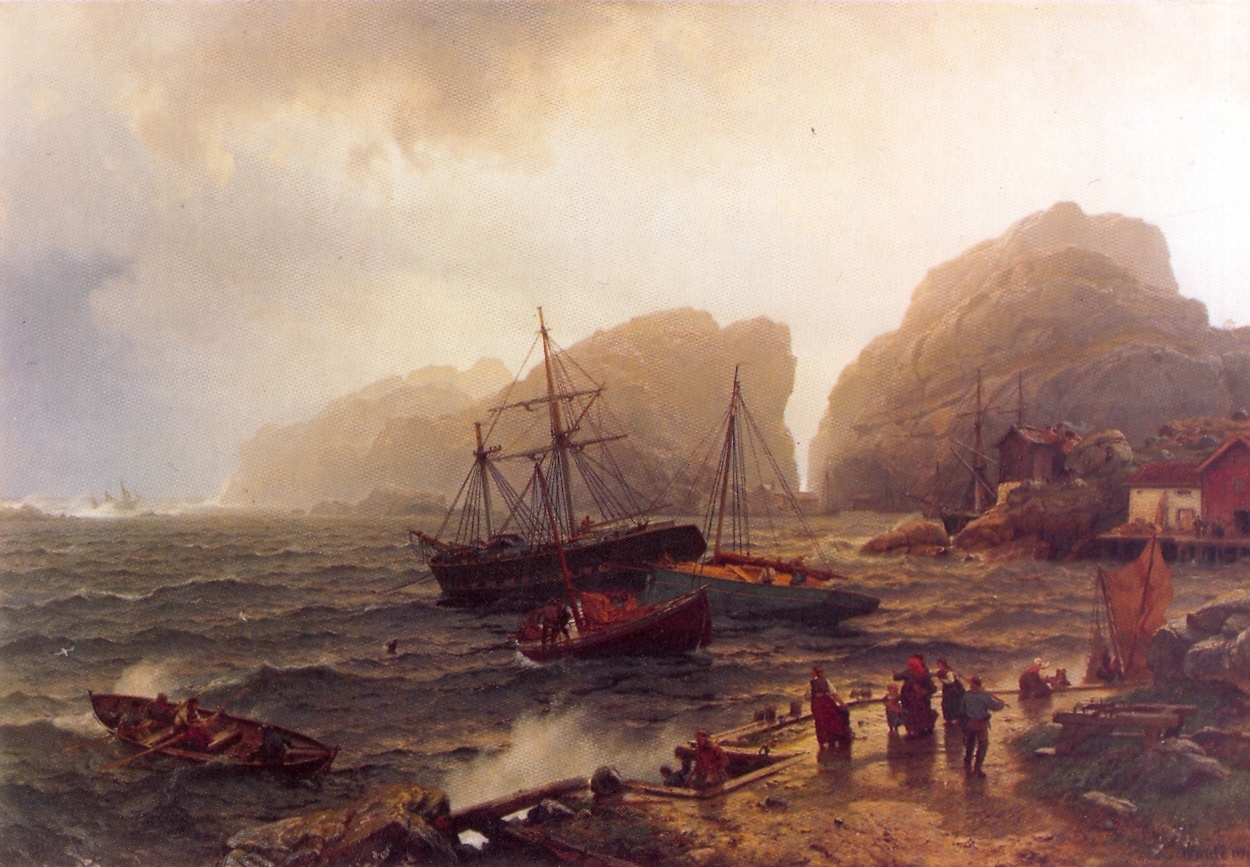This detailed painting depicts a historical European coastal scene, focusing on both the lively sea and the bustling shore. On the left side, the grey sea is filled with several boats and ships, battling waves as they make their way toward the brown, sandy shore on the right. Among four vessels nearing the shore, three are painted red and one blue, each carrying people, with boatmen visibly rowing. On the shore, a blend of men, women, and children stand watching the incoming boats. The shore is dotted with small houses, a flag, and a small port town extending into hills and mountains. In the background, rocky cliffs and dark and light clouds dominate the sky, complemented by the golden glow of the sun reflecting on the water. The scene seems to capture an era around the 1700s to 1800s, highlighting the significance of maritime activities with meticulous detailing of waves crashing onto the shore and the people amidst this dramatic seascape.